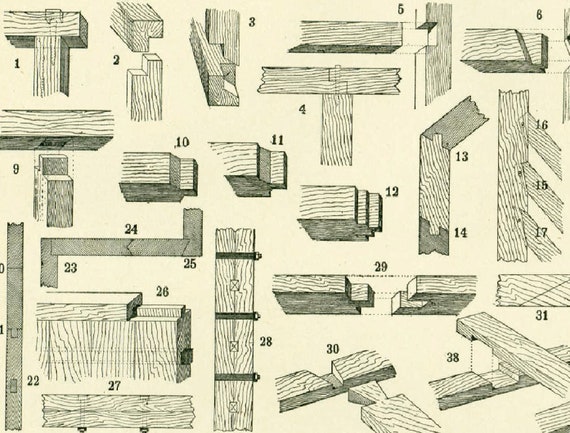This detailed pencil drawing on tan paper is a comprehensive diagram showcasing approximately 30 different types of woodworking joints, meticulously organized and rendered. Each joint is clearly numbered in black, though not all numbers from 1 to 38 are sequentially displayed, suggesting a partial view of the complete diagram. The artist presents a variety of joints, including dovetail, mitered, lap, butt, and corner joints, among others, used in constructing walls, headers, and footers. The detailed line work captures the wood grain and three-dimensional shapes of the various types of dimensional lumber, like 2x4s. This illustration resembles a technical guide from a carpentry or home construction reference book, offering a visually rich and instructive look at wood joinery techniques.